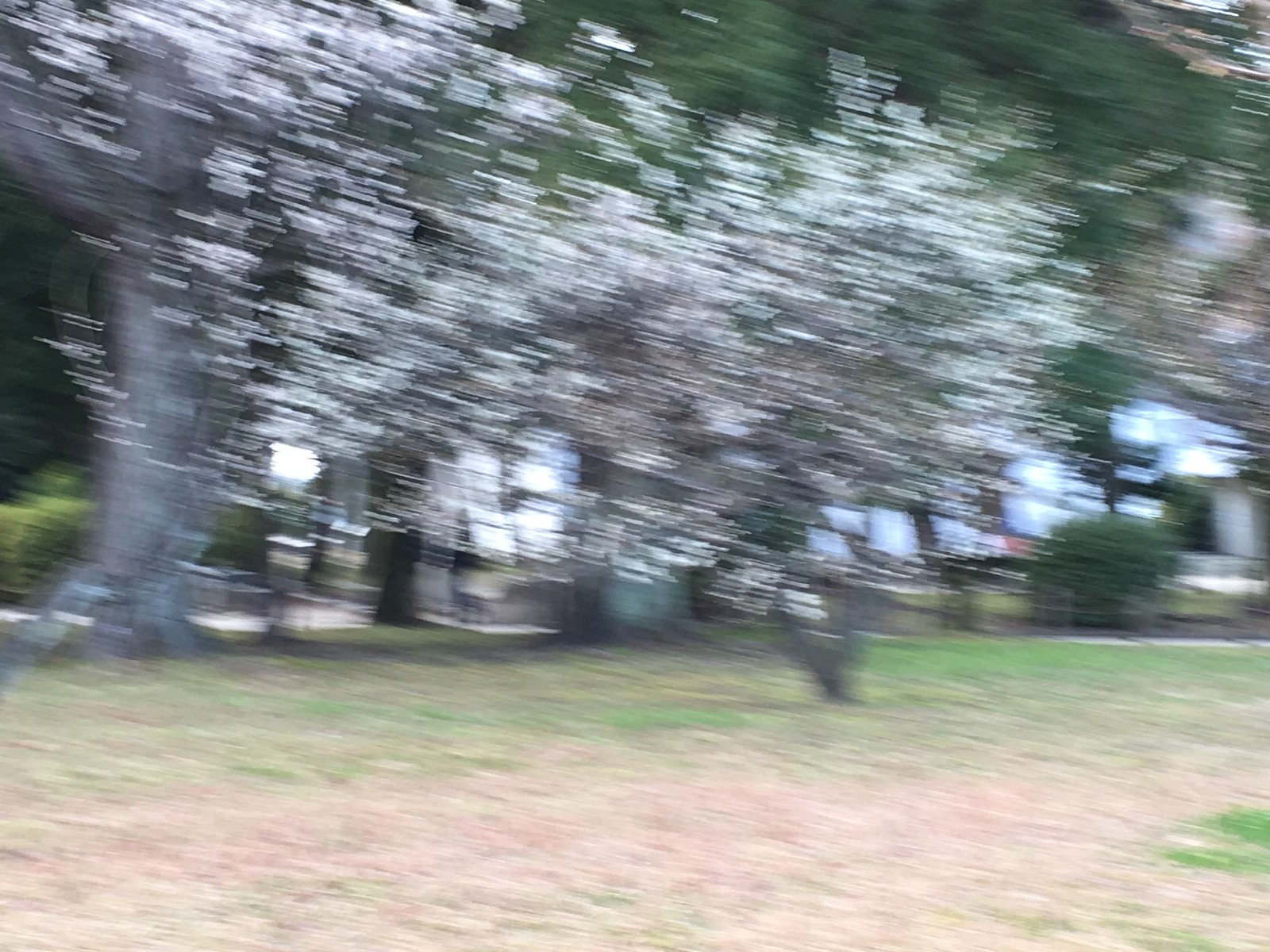This is a blurry photograph of an outdoor area that resembles a park. The bottom portion of the image shows a patchy, dirt-laden grassy field, where the grass appears trampled, revealing earthy yellows and beiges with sporadic green patches. Moving upwards in the image, there is a blend of more grass, dirt, and a small sidewalk, accompanied by a wooden fence. Above this, there are blurred trees and bushes, predominantly green, interspersed with white specks that could be flowering trees or motion blur artifacts. The trees' trunks show as a deep grayish color. At the top of the photograph, green leaves and a bit of blue sky are faintly visible amid the intense blur, giving the impression of motion.